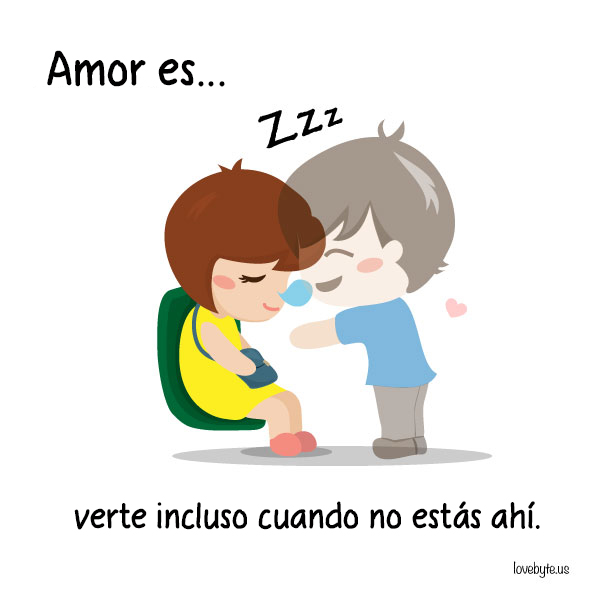The image is an illustration styled in animated graphics, set against a white background. In the center, a girl with short brown hair is depicted sitting on a green chair, apparently asleep with "ZZZ" above her head. She is dressed in a yellow dress and pink shoes, and she holds a small green purse in her hand. Beside her, slightly overlapping, is the semi-transparent figure of a boy with brown hair that has tan undertones. The boy is dressed in a blue shirt, grey pants, and brown shoes; he is depicted with a smile and rosy cheeks, reaching his hand out with a small heart floating near his head. Text on the image reads "Amor es verte incluso cuando no estás ahí," which translates from Spanish as "Love is seeing you even when you're not there." The bottom right corner of the image bears the attribution "lovebyte.us."